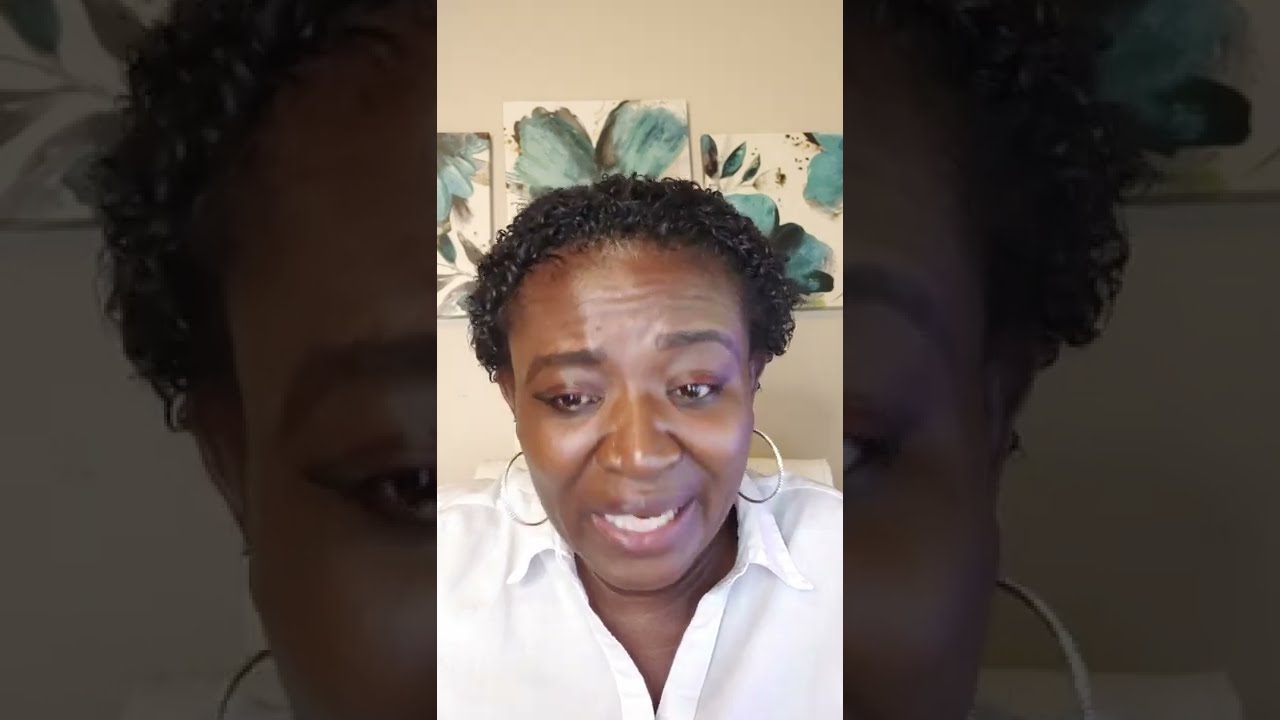The image is a triptych featuring a Black woman with short curly hair and gold hoop earrings. The left and right segments are darkened, each highlighting half of her face. In the left segment, we see the left half of her face and her earring, while the right segment shows the right half of her face and another earring, giving a mirrored effect. The central image is clear and shows the woman facing the camera with an astonished expression. She is wearing a white button-down shirt and appears to be speaking, possibly during a video or live stream. Behind her, three paintings with blue leaf-like designs are aligned in a row. The background and objects are predominantly tan, green, blue, gray, black, brown, and white, adding to the setting which suggests the image might be a screenshot taken from platforms like TikTok or Instagram Live. The overall composition and detail emphasize the woman's expressive face and the decorative background elements.